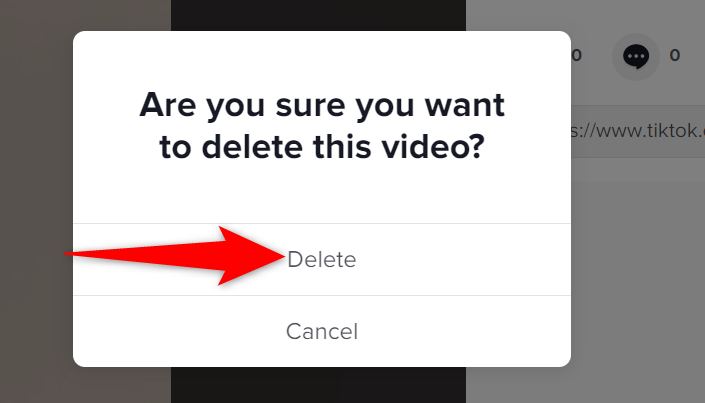In the image, we see the TikTok app interface, showcasing a screen for a video deletion confirmation. The background features a TikTok video that appears mostly black, displayed slightly at the top and bottom of the screen. 

At the top left corner, there is a comment icon with a label indicating zero comments. A URL for the video is partially visible, starting with "TikTok.com" followed by a forward slash and the username, although the full URL and username are not shown.

Prominently, a white pop-up appears in the center of the screen, containing text in black that reads, "Are you sure you want to delete this video?" Below this message, there are two options: "Delete" on the left and "Cancel" on the right.

A red, solidly filled arrow points to the "Delete" button, indicating where to press in order to proceed with deleting the video. The overall scene provides a clear guide for users on how to delete a video within the TikTok app, emphasizing the "Delete" option with the red arrow.